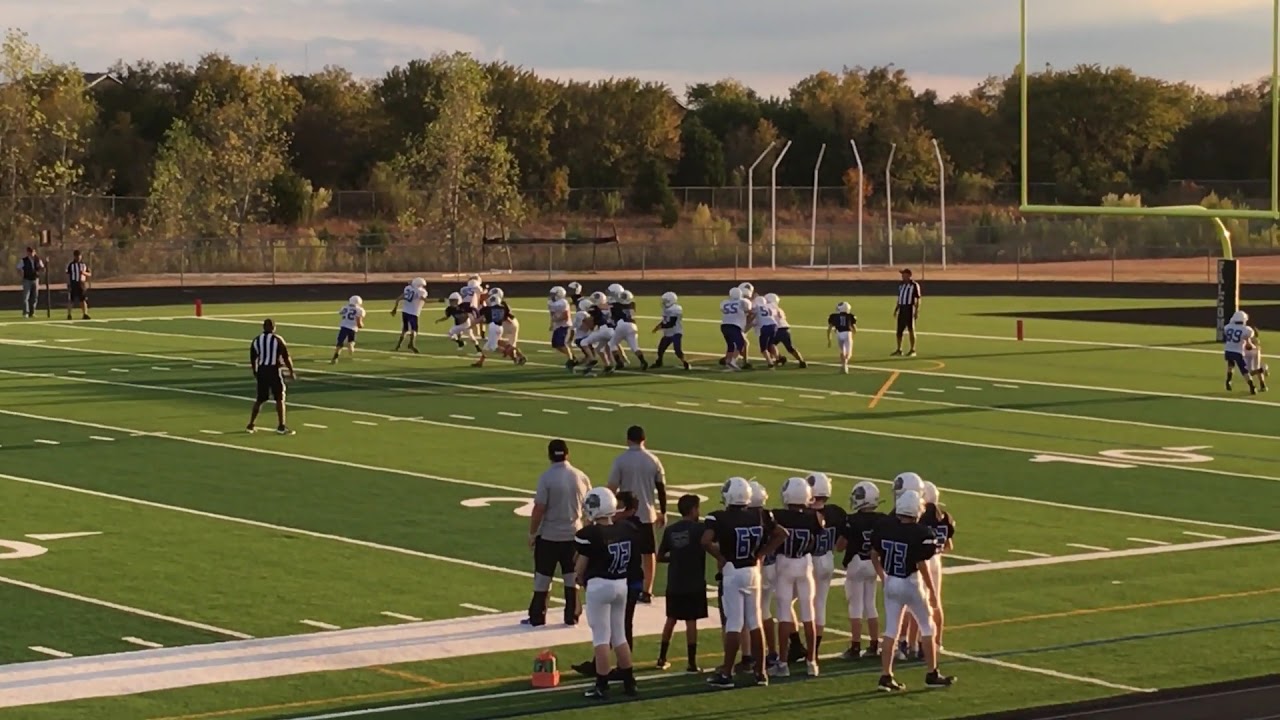In the image, a vibrant green football field is seen, prominently marked with white stripes and yard lines, including the 10-yard, 20-yard, and partially the 30-yard lines. At the center of the action are young football players engaged in a game near the 10-yard line. One team wears dark jerseys, white pants, and white helmets adorned with an emblem, while the opposing team is in white jerseys, dark pants, and also white helmets. Several referees dressed in black shorts and black-and-white striped jerseys can be observed on the field managing the game.

On the sideline, two adult men who appear to be coaches stand, with a group of about 10 players behind them, all dressed similarly in white pants, dark jerseys, and white helmets. A goal post, painted bright yellow, is visible in the background. Surrounding the field are green trees, and beyond the woods, a fence encloses the area. The sky above is a clear blue, dotted with a few white clouds, completing the scene with a touch of natural beauty.